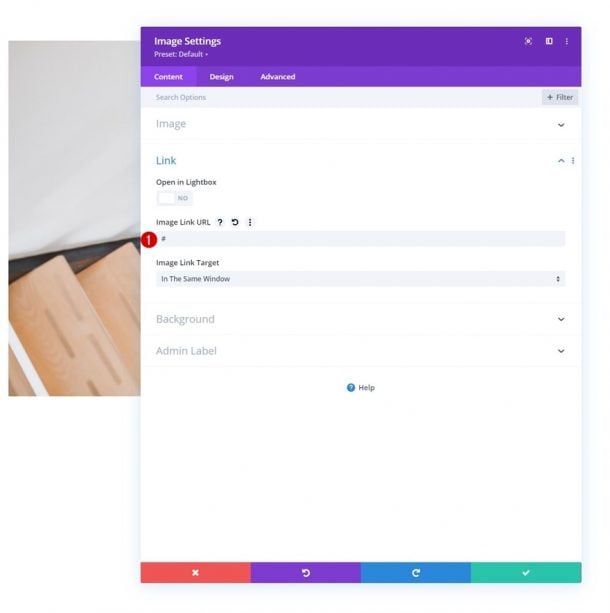The image displays a pop-up menu overlay on top of another website, likely related to web design or configuration settings. At the top, there's a purple strip labeled "Image Settings - Preset Default". Below this, there are three tabs: "Content," "Design," and "Advanced," with the "Content" tab currently active. The active tab shows multiple options including "Search Categories," "Image Link," "Open in Lightbox," and "Image Link URL." A notable detail is a small red circle with the number '1' next to the "Image Link URL" field, which also has a trio of vertical dots suggesting more options. This likely indicates a critical notification or step in a tutorial.

Further down, the interface lists additional fields such as "Image Link Target," with the option "in the same window," and "Background Admin Label." An information icon, represented by a small circle with a question mark, suggests help or additional information is available.

The background of the page is predominantly white with some gray elements, indicative of a clean UI design. At the bottom of the interface, there are various colored blocks representing different actions, including a red X (close or cancel), a purple arrow (back), a teal arrow (forward), and a green checkmark (accept or confirm). Given the presence of the red circle with the number '1', this interface likely belongs to an interactive tutorial or a learning tool guiding users through image link settings within a web design application.